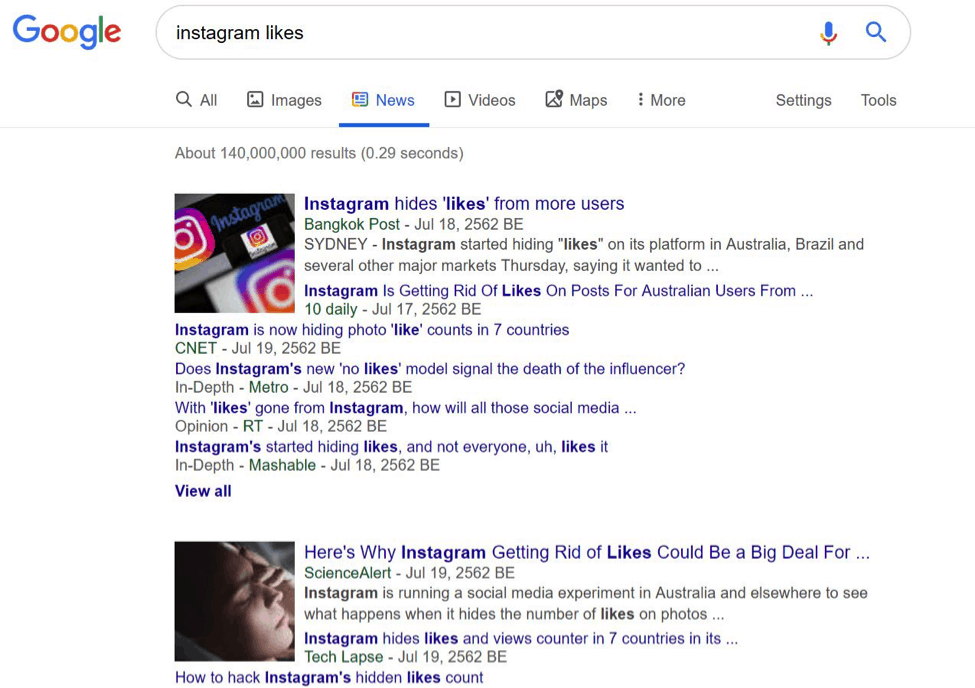The image depicts a Google search results page with the query "Instagram likes" entered. In the top-left corner, the colorful Google logo is visible, featuring the iconic capital 'G' in blue, followed by a red 'o', a yellow 'o', a lowercase green 'g', a lowercase blue 'l', and a lowercase red 'e'. The Google search bar at the top of the page includes a microphone icon on the left and a magnifying glass icon on the far right.

Below the search bar, multiple search results are listed. The first search result is highlighted in bold blue text and reads "Instagram hides likes from more users - Bangkok Post." Adjacent to this result is a small, square icon depicting the Instagram logo. Notably, the date on the search result is given as "July 18th, 2562 BE."

Underneath the title of the first search result, the snippet reads: "Sydney. Instagram started hiding likes on its platform in Australia, Brazil, and several other major markets Thursday."